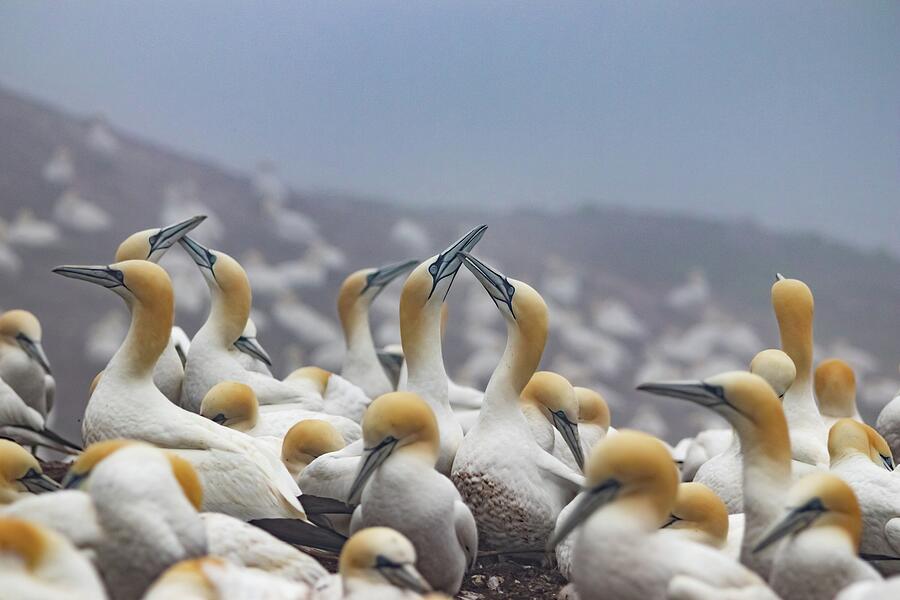This image showcases a flock of small, identical birds arranged predominantly across the lower portion of the frame. The majority of these birds are only partially visible, with focus on their heads and upper bodies. A few birds in the distance, especially the one in the center, are more distinguishable. These birds display a consistent color pattern: a gray lower body, primarily white plumage, a white neck underside, yellow on the top of the head extending down the back of the neck, a gray beak, and striking black eyes. The orientation of the birds varies, with many facing left, some right, and others showing their backs by facing directly away. The backdrop features a blurry mountainous landscape under a light blue sky, adding depth to the scene.